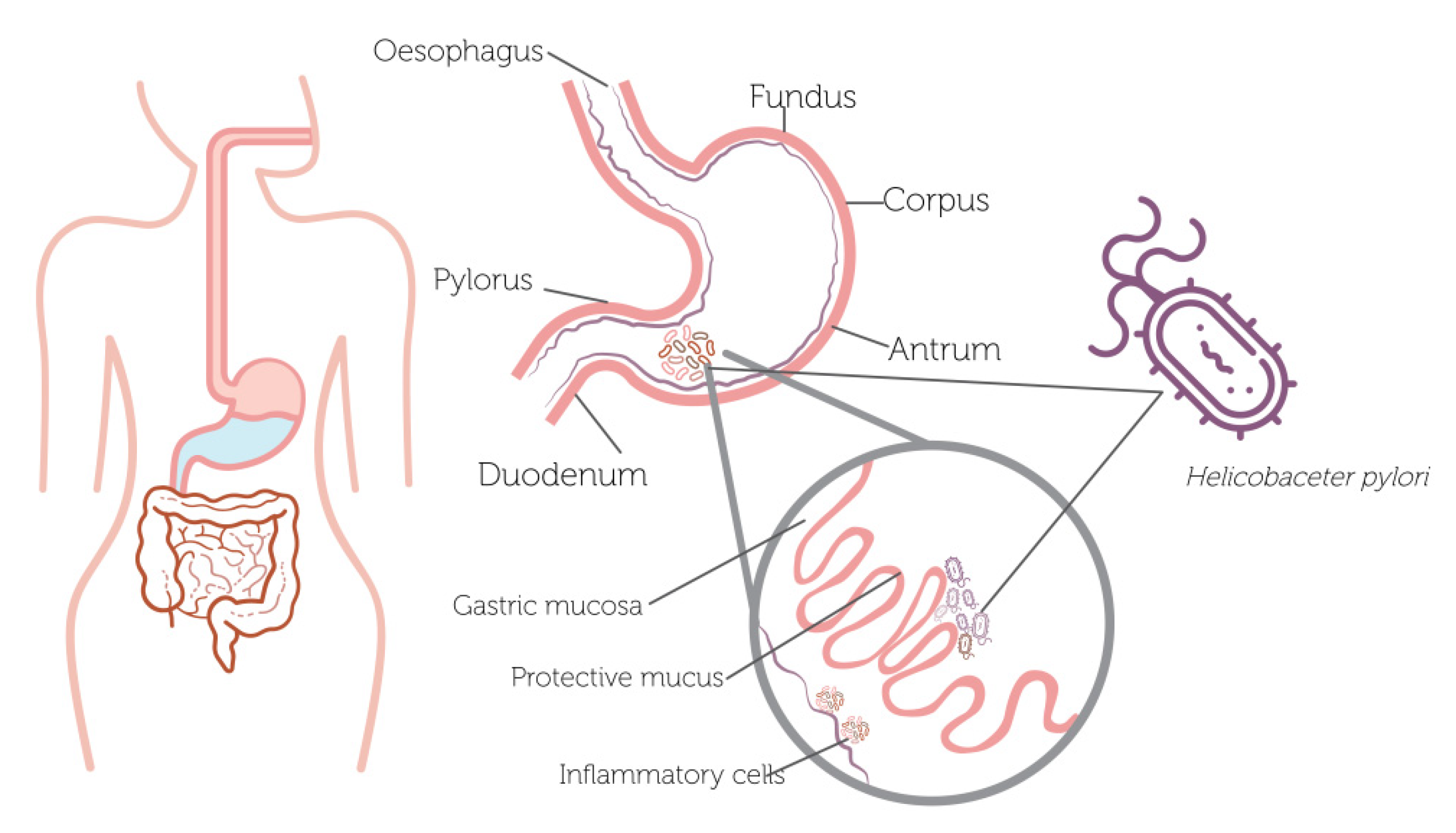The image depicts a detailed diagram of the human digestive tract on a white background. On the left side, there is an outline of a figure, which could be male or female. The figure's internal anatomy is shown, featuring a tube descending from the mouth into the esophagus, leading down to a pink stomach, which is partially filled with blue representing water, and the intestines, outlined in red. On the right side, a more detailed blowup showcases various parts of the digestive system: the esophagus, fundus, corpus, antrum, pylorus, and duodenum. Additionally, there is an enlarged depiction of a purple, bacteria-like object identified as Helicobacter pylori, alongside another close-up showing the gastric mucosa, protective mucus, and inflammatory cells, with each component annotated in black text. The color scheme includes pink, black, purple, brown, and light blue, contributing to the informative and visually distinct presentation of each element in the diagram.